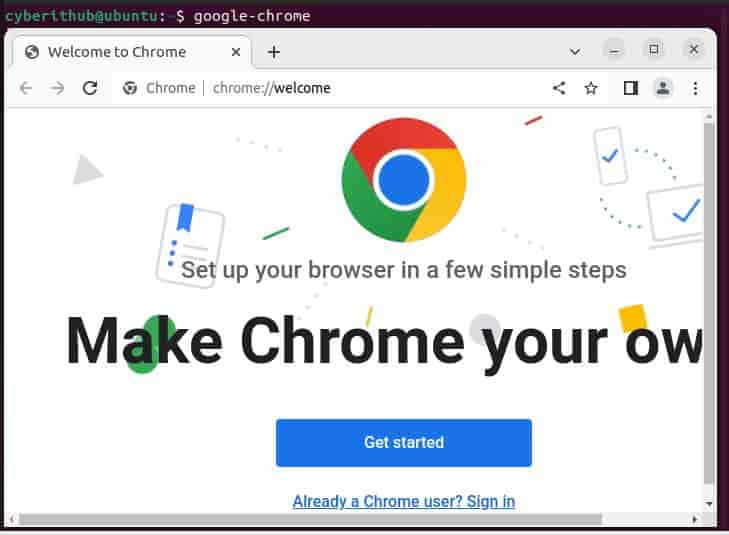The image depicts a screenshot of a Google Chrome browser running on a Linux system, specifically Ubuntu. At the top left corner, the terminal prompt shows "cyberthub@ubuntu:~$ google-chrome," indicating the user's environment. The text "cyberthub@ubuntu" is highlighted in green, contrasting with the white text of the rest of the command, all set against a purplish background. 

The browser itself displays only one tab titled "Welcome to Chrome" in black text. The URL bar reads "chrome://welcome" with the word "welcome" in a darker black. At the top right corner of the browser interface, the typical control icons for minimizing (a dash), maximizing (a square), and closing (an X) the window are visible.

In the main window of the browser, there is a welcome message that reads "Set up your browser in a few simple steps." Above this text is the Google Chrome logo, prominently featuring its iconic colors: red, yellow, green, blue, and white. At the bottom center of the screenshot, the words "Make Chrome your own" are displayed, followed by a blue rectangular button with the text "Get Started" in white, inviting the user to begin customizing their browser.